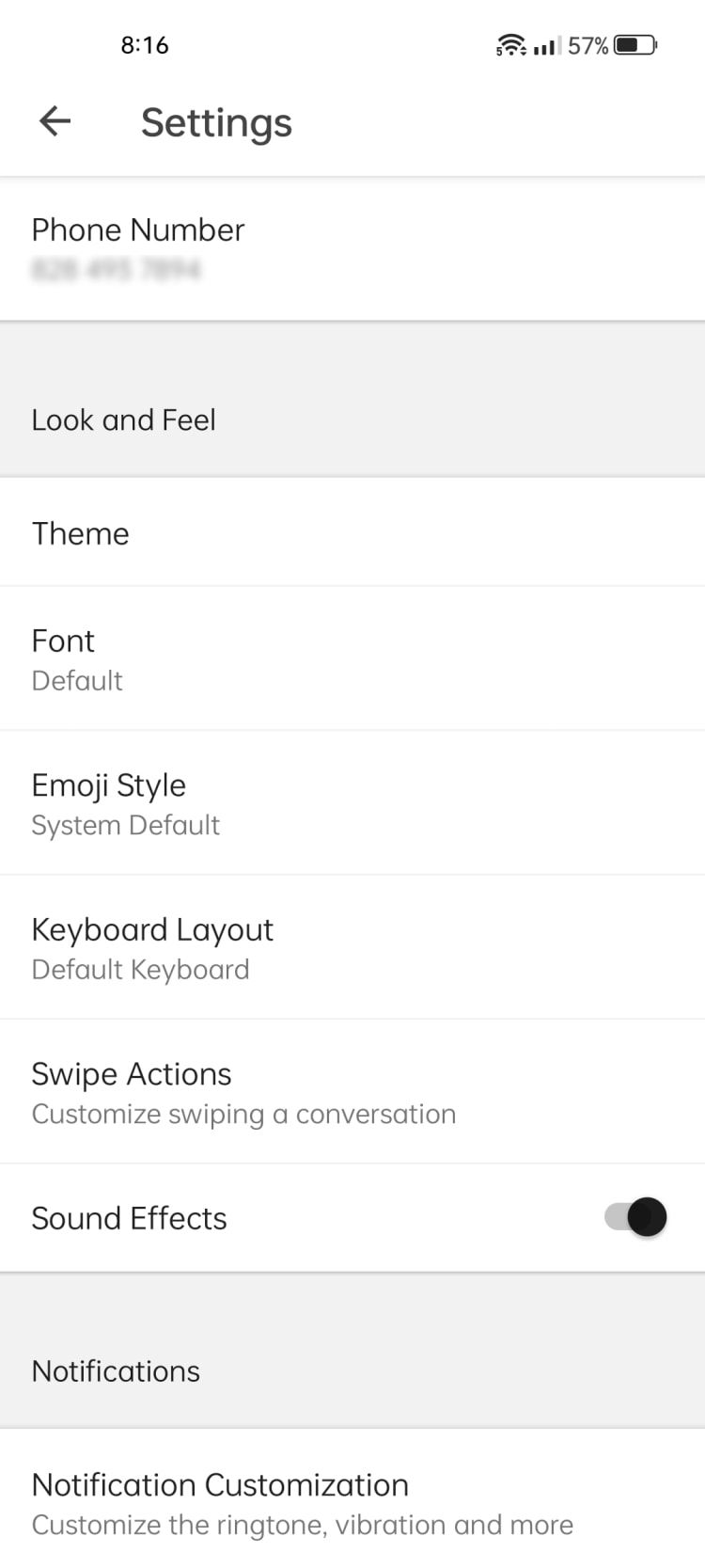Caption: 

A screenshot captured on a smartphone displays a mobile settings menu against a white background with black text. At the top-left corner, the time is visible, while the top-right corner shows the battery percentage, battery icon, network signal icon, and WiFi icon. Directly below, an arrow pointing left indicates a "Back" option next to the "Settings" title.

Further down, a blurred-out phone number is partially visible. A grey band titled "Look and Feel" divides the sections, under which options like "Theme," "Font," and "Emoji Style" are listed. The "Emoji Style" is set to "System Default," while the "Font" and "Keyboard Layout" are both indicated as "Default." Additionally, "Swipe Actions" is described with the text "Customize swiping in conversation."

The "Sound Effects" switch is turned on, as denoted by a black circle within the toggle icon. Another grey band labeled "Notifications" follows, beneath which "Notification Customization" with grey text reading "Customize" appears, along with other options for managing ringtone, vibration, and more.